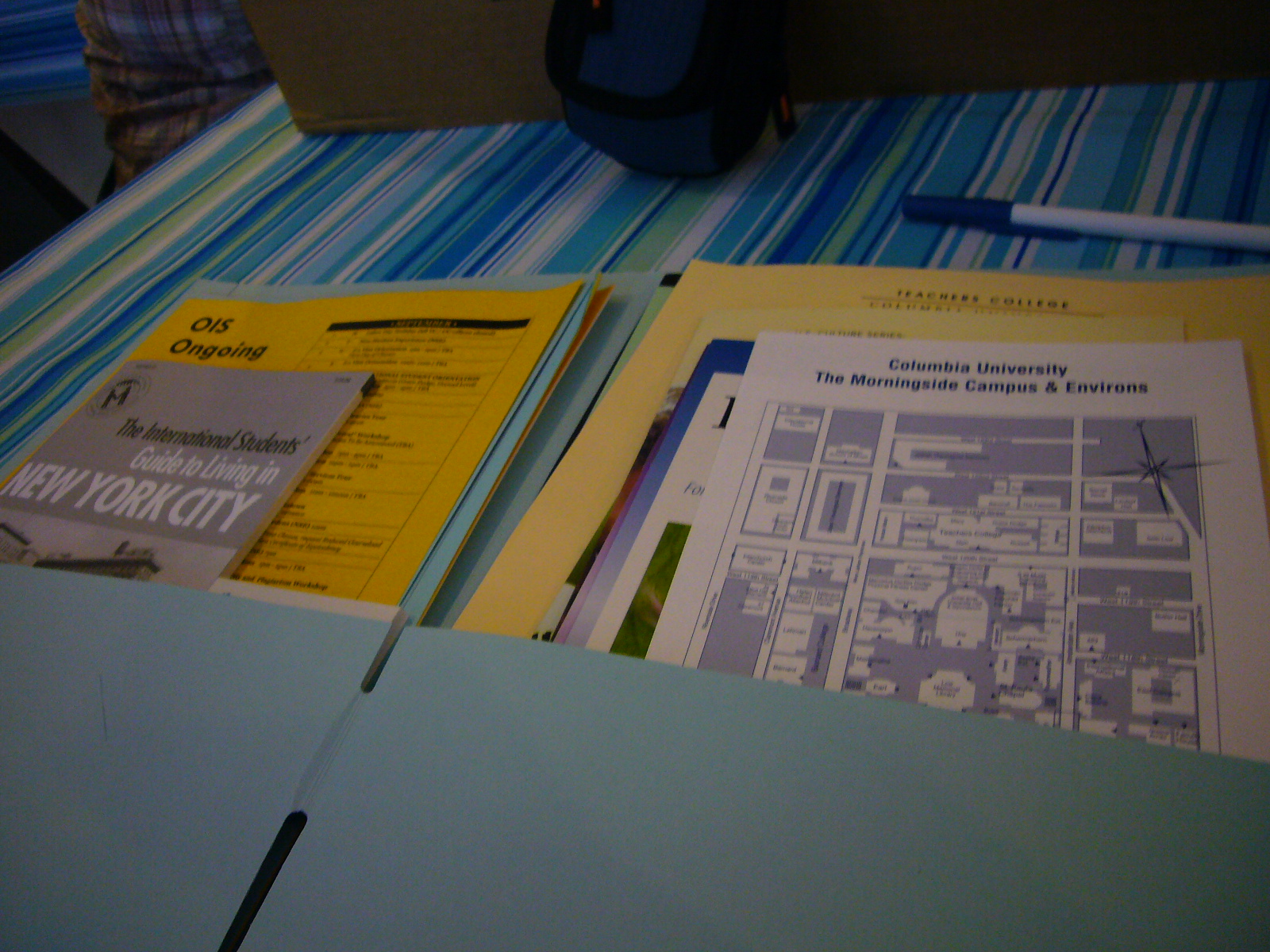This is a detailed photograph of a college student's open folder, which is situated on a table covered with a striped cloth in shades of blue, green, white, dark blue, and yellow. The pale blue folder has two pockets and contains various papers and brochures. In the left pocket, there is a conspicuous International Students Guide to Living in New York City and a yellow page whose text is unreadable. The right pocket holds a campus map of Columbia University's Morningside Campus and additional, unidentified pamphlets. Positioned above the folder on the table is a blue ballpoint pen with a cap. This setting likely marks the beginning of the student's academic journey at Columbia University, possibly on their first day of preparation.